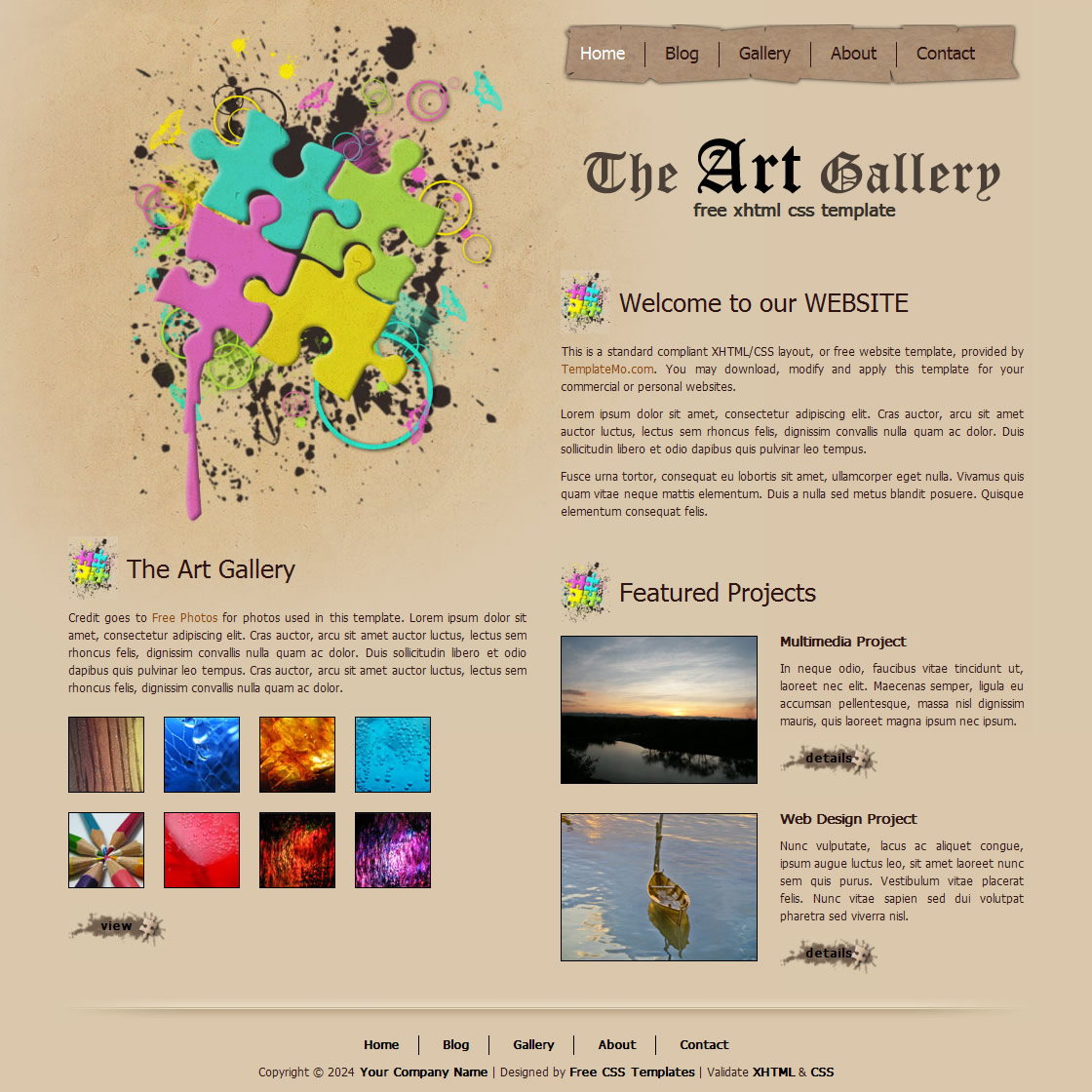The image is a detailed screenshot of a webpage with a light brown, almost tan, background. The top right corner features navigation links labeled "Home," "Blog," "Gallery," "About," and "Contact." The "Home" page is highlighted in white, indicating it is the current page. Just beneath these tabs, black text reads “The Art Gallery Free XHTML CSS Template.” Below this, a welcoming message says, “Welcome to Our Website,” accompanied by a small image of four puzzle pieces in blue, green, yellow, and purple.

The webpage is divided into two main sections. On the left, under “The Art Gallery,” there is credit text that states the photos come from “Free Photos.” The text also includes some placeholder "Lorem ipsum" text. Additionally, there are eight square images at the bottom of this section, including abstract designs and an image of color pencils arranged in a circle.

On the right side, labeled "Featured Projects," there are headings for "Multimedia Projects" and "Web Design Projects," each with corresponding images showcasing examples of these projects. 

At the very bottom of the page, the navigation links “Home,” “Blog,” “Gallery,” “About,” and “Contact” are repeated in black text. The footer also includes a copyright notice, “© 2024 Your Company Name,” and a note mentioning “Designed by Free CSS Templates,” with validation for XHTML and CSS.